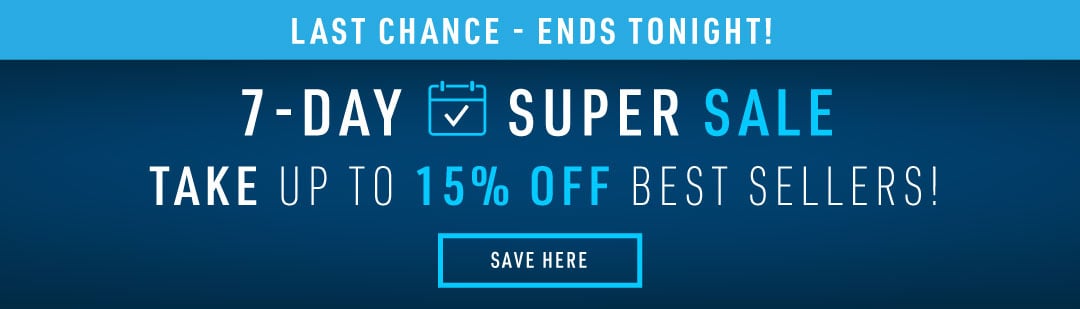The image is a horizontal rectangular banner that prominently features an ad. The top portion of the banner stretches across its entire width and is colored in a gradient of light blue and white. It contains the bolded text: "Last chance. Ends tonight!" in dark blue.

Below this section, the rest of the banner has a dark blue background. The phrase "Seven Days" is displayed in bold white text, accompanied by a calendar icon with a check mark. Below this, bold text in varying colors reads: "Super Sale, Take up to 15% off Bestsellers." The words "Super Sale" and "15% off" are in blue, while "Take up to" and "Bestsellers" are in bold white.

At the bottom right corner of the banner, there is a call-to-action button. This button is surrounded by a light blue border and has a dark blue fill. Inside the button, the text "Save Here" is written in white.

The banner uses a consistent color scheme of white, light blue, and dark blue, with no other colors or details that specify the products on sale or the website it is advertising. The overall design suggests that this banner is likely intended for placement on various websites to attract attention with its sense of urgency and bold, contrasting text.